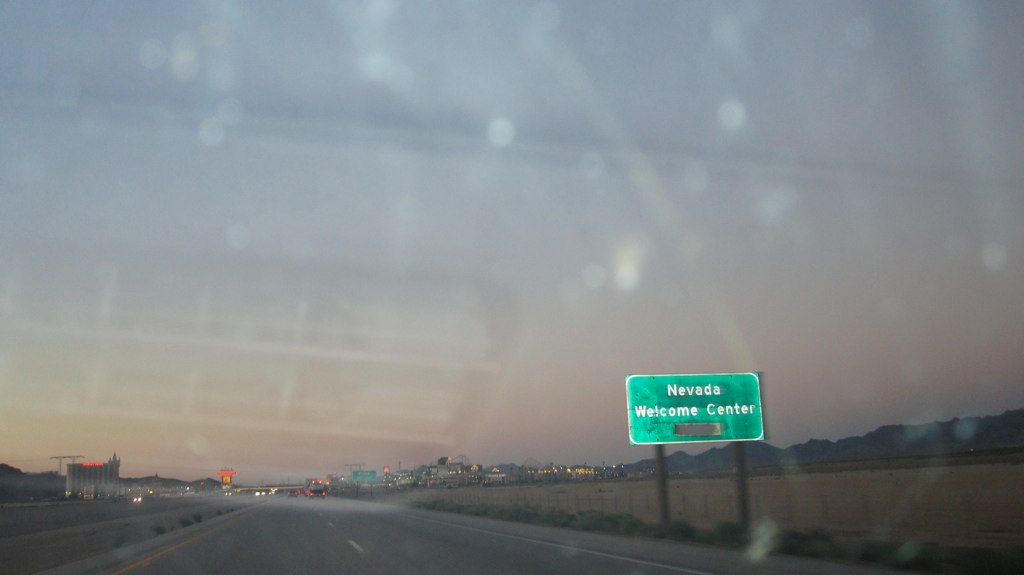A photograph taken from inside a vehicle captures a scene at dusk or dawn, possibly through a rain-streaked or dusty windshield. The sky is painted in shades of purple and pink, casting a dim light over the landscape. The vehicle is traveling on a two-lane road, heading towards the Nevada Welcome Center, as indicated by a green highway sign with white lettering, mounted on two metal poles on the right side of the road. In the distance, the road leads to an area filled with businesses and hotels, their lights glowing softly in the early or late hours. Dry, brown fields stretch out on either side of the road, with clusters of trees standing beyond them. The headlights of oncoming cars illuminate the way down the highway, creating a serene yet vibrant scene as Nevada welcomes the travelers.